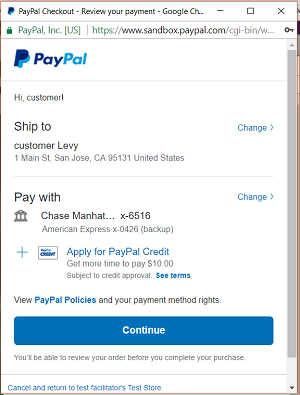The image displays a PayPal checkout window for reviewing a payment. The central focus is on the PayPal interface, which features a "Review your payment" section. The greeting "Hi Customer" is visible, followed by shipping information: "Ship to Customer Levy," located at "1 Main Street, San Jose, California." The payment method highlighted is "Chase Manhattan" with the card number partially obscured. An alternative option to "Pay with Apple Credit" is also available.

Various actions and options are presented, including:

- A "Change" button for modifying the shipping address.
- A link to view PayPal policies.
- A prominent blue "Continue" button at the bottom of the window.
- A link to "Cancel and return to Test Facilitator's Test Store."

Additionally, there's a mention of a PayPal Credit offer, stating: "Get more time to pay $10, subject to credit approval." In the background, a few pixels hint at an additional, indistinct element on the right side of the image. The items being purchased are not specified.